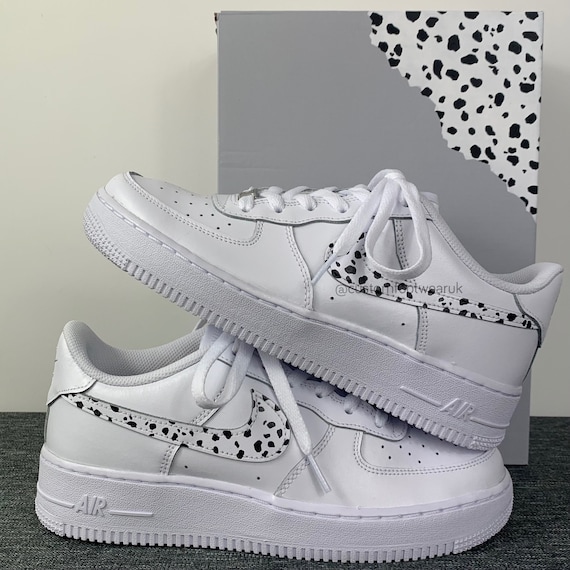The image features a white background, resembling a wall, with a gray, carpeted floor. A gray box is present, notable for its black and white Dalmatian print on the upper right-hand corner. The primary focus of the image centers on a pair of Nike Air tennis shoes. These shoes are predominantly white, except for the Nike logo, which is adorned with the same black and white Dalmatian print. The shoes are arranged with one on top of the other; the bottom shoe points to the right, while the top shoe points to the left. There is also a watermark on the top shoe that reads "At Custom Footwear, UK," indicating that the shoes have been customized and are part of a promotional display for bespoke Nike Air footwear.